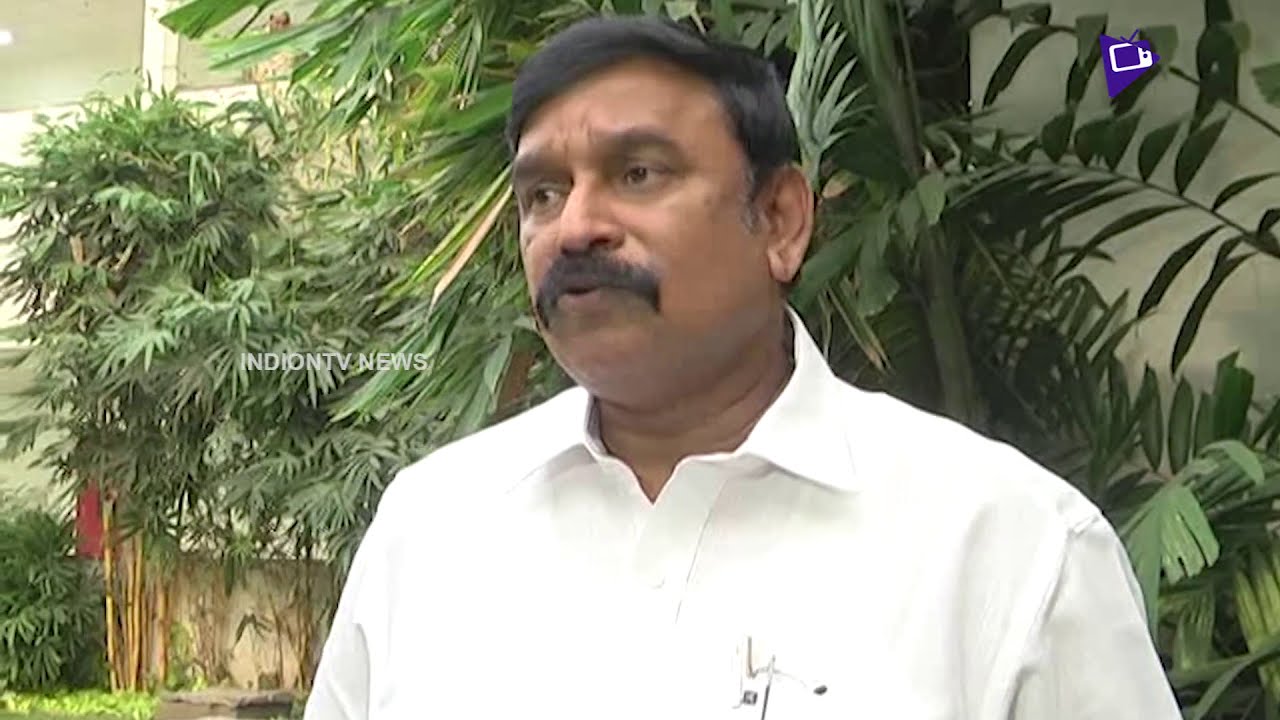This photograph depicts a middle-aged Indian man with short black hair and a mustache, wearing a classic white button-down shirt complete with a pen protector and a pen in his chest pocket. The man is positioned against a backdrop of lush, tropical-style plants, including palm trees, which partially obscure a white building in the background. He appears to be engaged in conversation, looking off to his left as if being interviewed. Supporting this context, watermarked white text on the image reads "Indian TV News." Additionally, a blue triangle with a white television icon is visible in the upper right corner, further indicating that this scene is part of a news interview or broadcast.